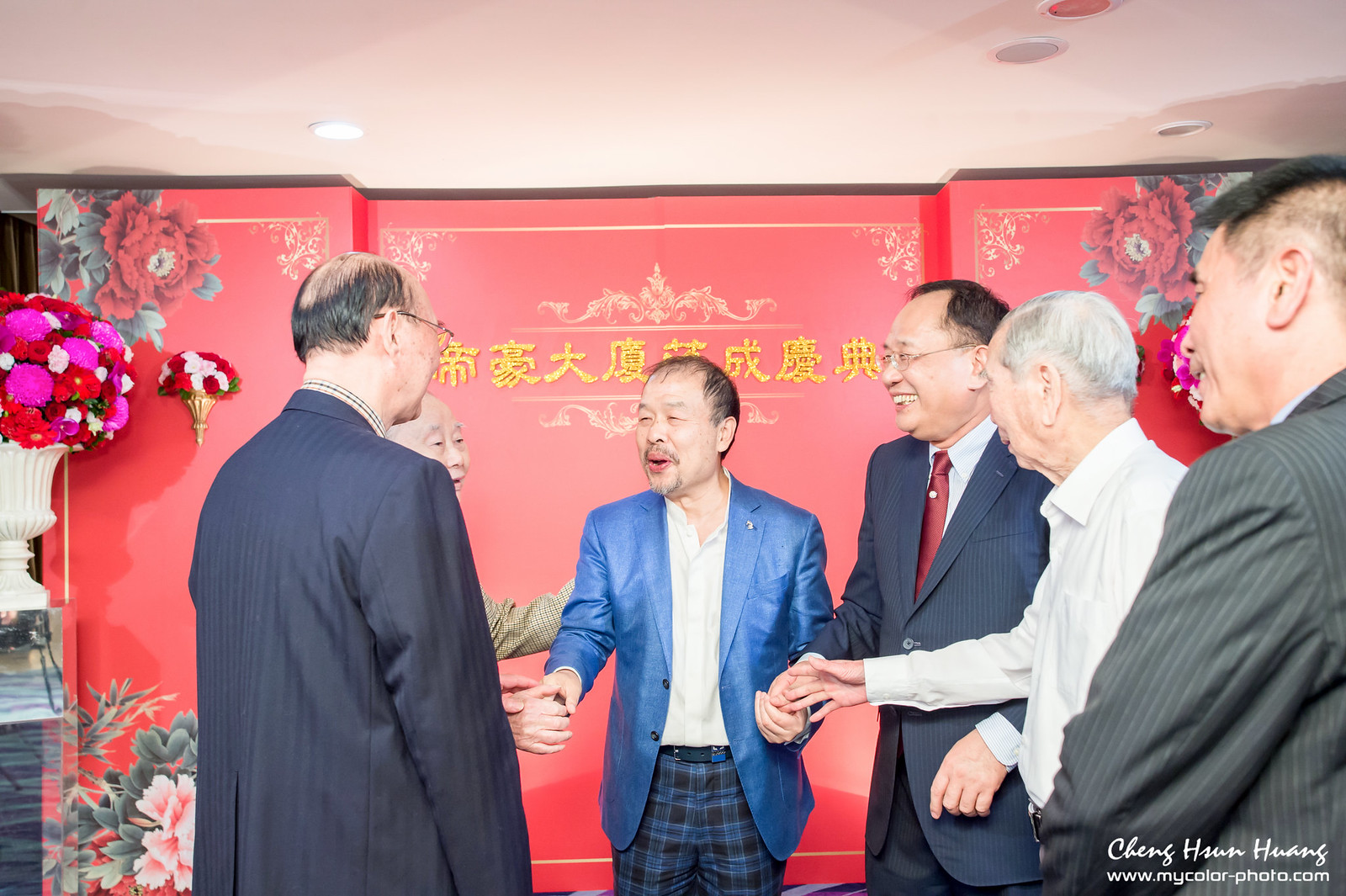This is a detailed photograph capturing a group of six elderly Asian men, seemingly in their 70s, standing in a semicircle and holding hands. The man in the middle stands out with his plaid pants, a light blue jacket, and a white dress shirt. To his right, two other men are dressed in suit coats, while the man directly to his left is older and clad in just a white dress shirt. The far left features another man in a suit, and next to him, only the head of the last man is visible. The setting appears to be an indoor space with a striking red wall adorned with ornate floral designs and large gold Chinese characters. Adding to the decor, there are white vases perched on pillars, each overflowing with large bouquets of red, white, and pink flowers. The bottom right corner of the image is marked with "Changsangheungcolorphoto.com," indicating the photographer or studio.